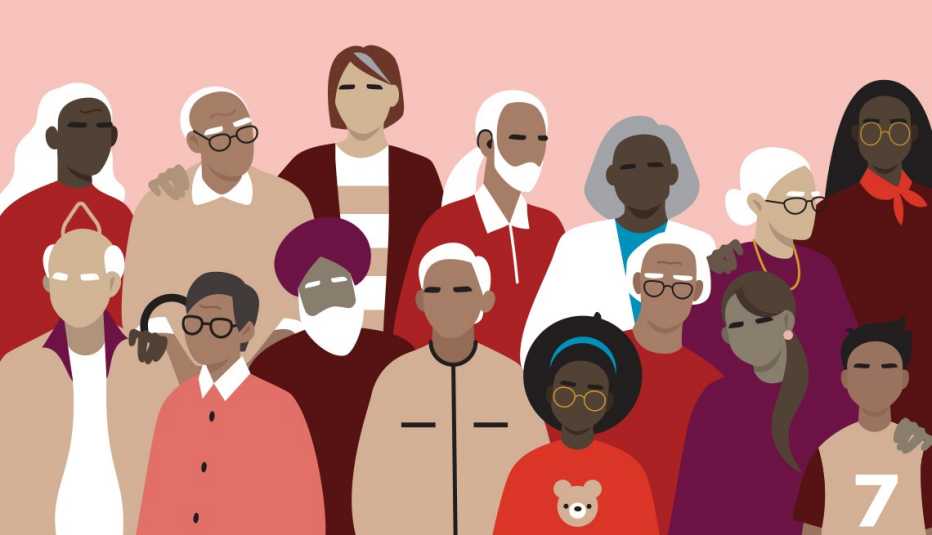This digital drawing features a diverse group of people arranged in two rows against a light pink background. The top row includes seven individuals: a Black woman with blonde hair in a red shirt, an older man with gray hair and glasses in a tan shirt, a woman with short reddish hair in a striped shirt and burgundy sweater, a man with long white hair in a ponytail and a gray beard in a red shirt, a person of indeterminate gender with gray hair in a white coat and blue t-shirt, an older woman with her gray hair in a bun, glasses, and a burgundy shirt with a necklace, and a Black woman with long black hair, glasses, and a burgundy shirt with an orange tie around the neck. 

The front row consists of eight individuals: an older balding man with gray hair, wearing a tan jacket and a burgundy collar, a man with dark hair and glasses in a pinkish shirt with black buttons, a man with a gray beard and turban in a burgundy shirt, a man with gray hair and black eyebrows in a tan shirt with two pockets, a Black woman with an afro, a blue headband, and an orange shirt with a teddy bear face, an older man with gray hair and glasses in a red shirt, a woman with long hair in a ponytail with pearl earrings in a red shirt, and a young boy with black hair and black eyebrows in a tan jersey with the number 7. Many of the characters rest their hands on the shoulders of the person next to them, and none of them have visible eyes or mouths, emphasizing their outlines, hairstyles, and clothing.